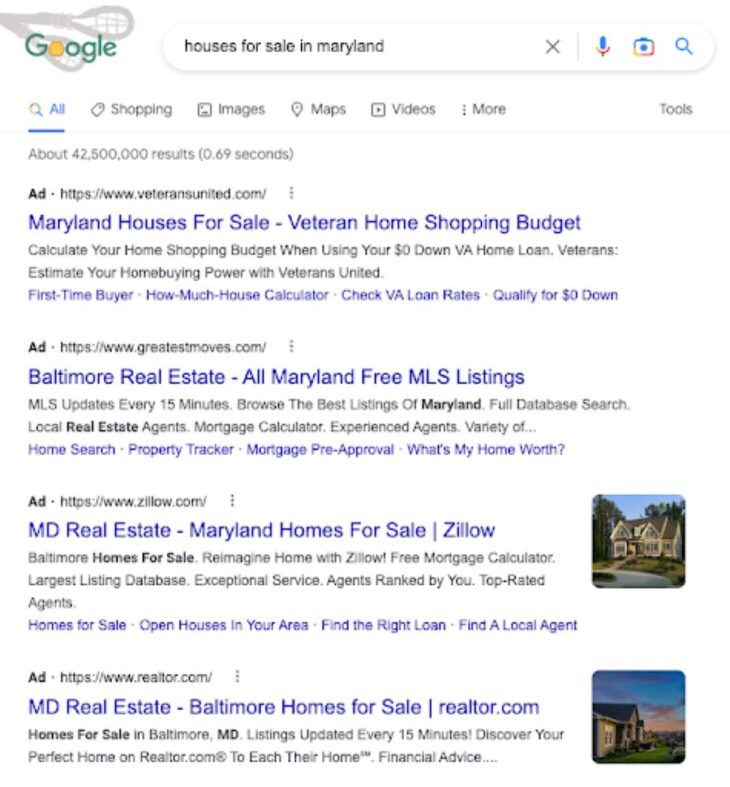A cropped screenshot of a Google search page is displayed, featuring a special Google Doodle at the top left corner. The Doodle includes a gray clipart image of crossed lacrosse sticks behind the word "Google," which is written in green text, with the first "O" depicted as a yellow ball. To the right of the Doodle is a search bar with the query "houses for sale in Maryland" written in a light gray font.

Below the Doodle and search bar are the search results, displaying four advertisements. Each entry is prefixed with the word "Ad" in bold black letters on the top left. Next to the "Ad" label, each result includes a link followed by the headline for the respective listing. 

The first ad lists "Maryland houses for sale, veteran home shopping budget," including several hyperlinks underneath. The second ad is from greatmoves.com. The third ad is from Zillow and features a thumbnail image to the right of the listing. The final ad is from realer.com, which also includes a thumbnail image to the right of its listing.